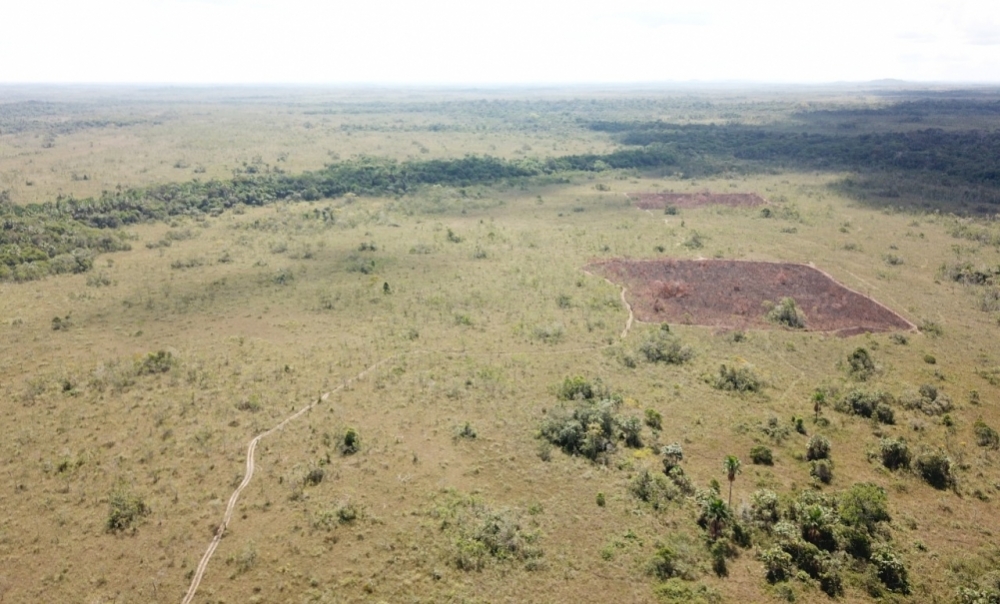The image depicts a high-level view of a vast, flat countryside landscape. The main features include a narrow road that starts from the bottom left, winding its way towards the upper left, culminating near two brown squares that suggest areas of cleared land or possibly farmland. The colors dominating the scene are gradients of green from the various shrubs and trees scattered throughout the image, interspersed with the brown hues of the dirt and the cleared plots. The foreground showcases a dense concentration of green foliage, particularly in the bottom right, while the upper portion of the image is predominantly occupied by more trees stretching across the horizon. The horizon itself is a pale white, devoid of any structures, people, or animals, emphasizing the openness and solitude of the landscape, reminiscent of a prairie or untended farmland.